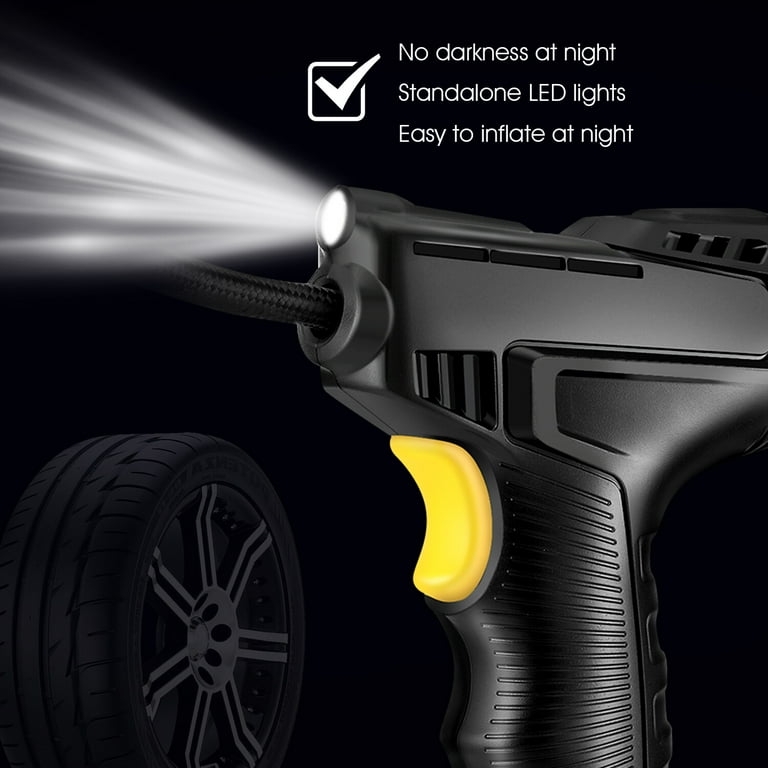The image features a handheld tire inflator prominently positioned against a solid black background. In the bottom left corner, a black tire with a dark gray rim is partially visible, subtly anchoring the scene. The tire inflator itself, positioned centrally and to the right, boasts a practical design with ergonomic indentations on the front-facing grip, ensuring ease of handling. A distinctive yellow trigger button is situated on the grip, adding a pop of color and functionality. Extending from the front of the device, a long black cord is clearly visible, hinting at operational convenience. Additionally, a bright white LED light is integrated at the front, underscoring its utility. At the top of the image, the text reads: "No darkness at night. Stand alone LED lights. Easy to inflate at night," highlighting the inflator’s night-time usability.